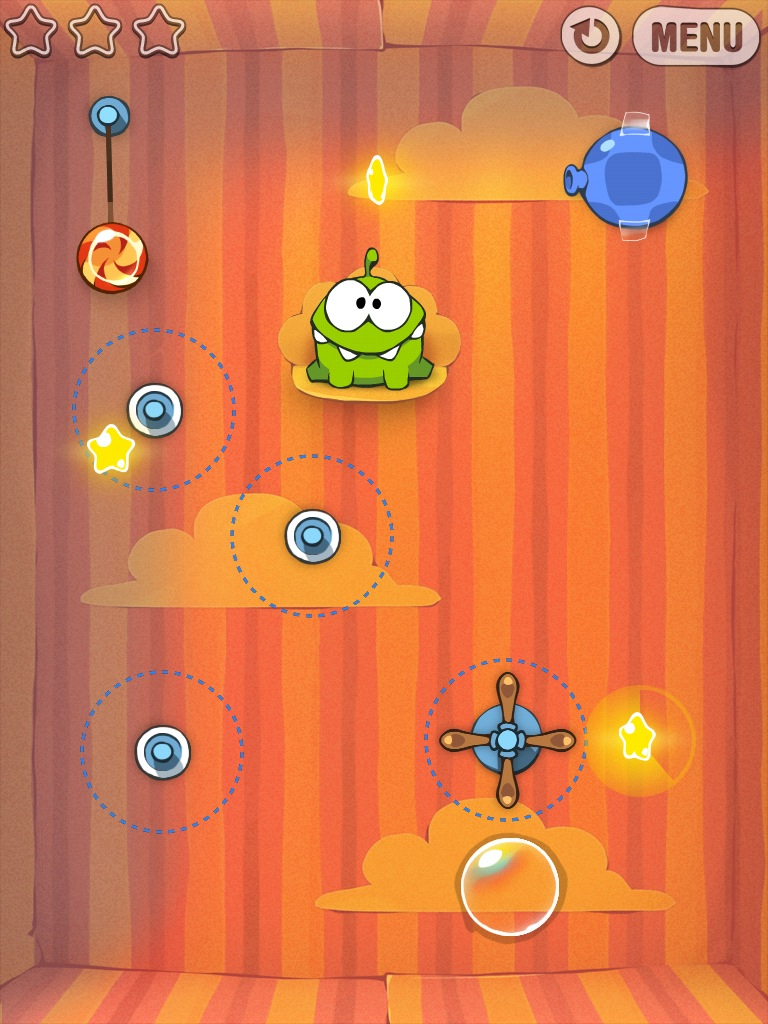This image is a vibrant, cartoonish screenshot of a mobile game displayed in portrait mode. The scene is dominated by a lively, green frog-like character or possibly a dinosaur, featuring two big googly eyes pointed inward and four prominent teeth. The background is a warm, visually engaging pattern of orange, yellow, and red stripes, giving it a wallpaper-like quality enhanced with orange clouds.

In the top left corner of the screen, there are three star icons, typical of mobile games to indicate performance levels, with three stars likely representing perfection. The UI also includes a redo button in the top right corner, designed as an arrow, and a menu button nearby, both of which are white with transparent backgrounds. 

The game environment is filled with playful objects including bubbles, stars, a lollipop, and a balloon taped to the top right of the screen. There are also yellow clouds and a distinctive spinning propeller located centrally. Below the main character, which appears just above the center of the image, are three dashed circles—one containing a propeller-like object and the other two empty, suggestive of interactive gameplay elements. The colorful, childlike design establishes a fun and engaging atmosphere consistent with mobile arcade games.